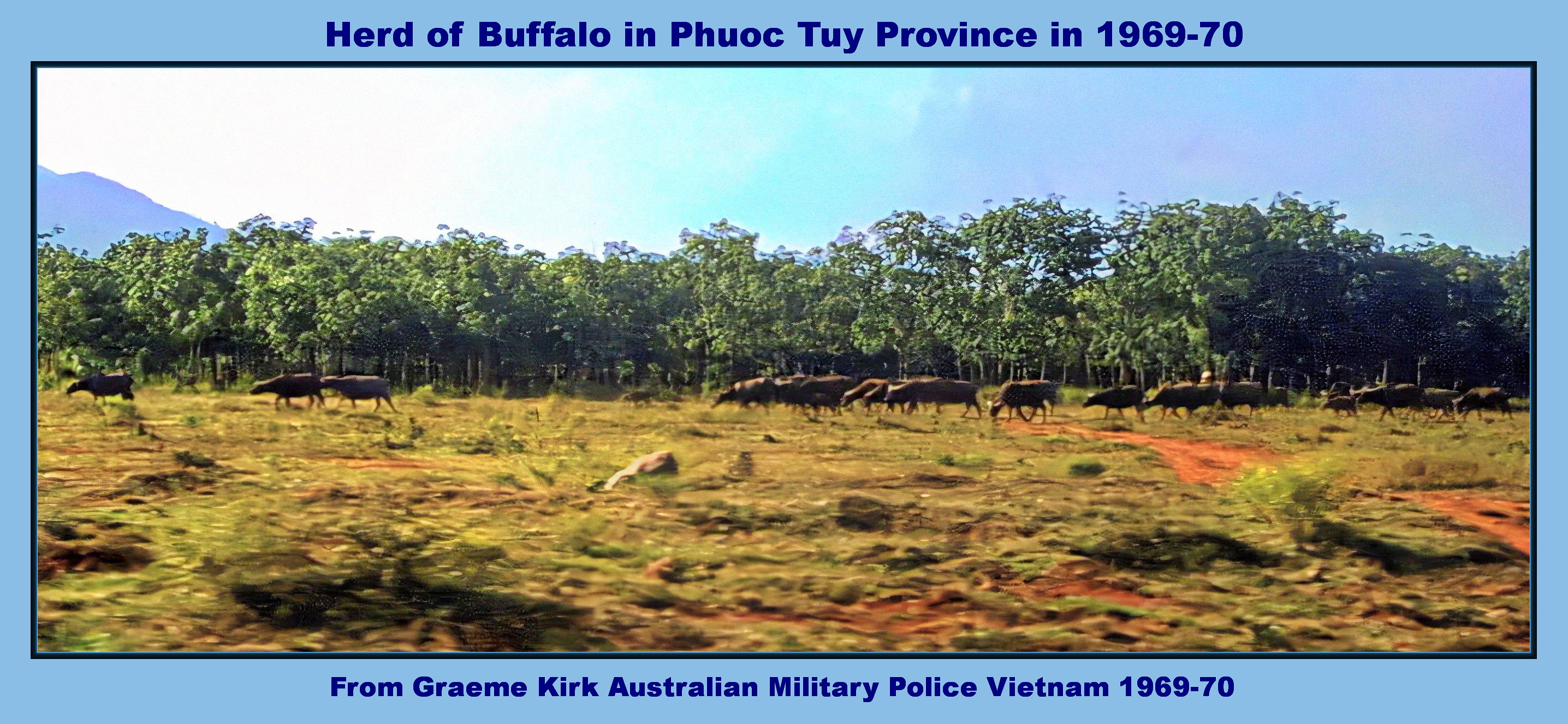The image portrays a widescreen panoramic view of a herd of buffalo in Phuoc Toi Province, Vietnam, dating back to 1969-70. The picture is encased in a light blue border with an additional black inner border. At the top, in dark blue text, it reads "Herd of Buffalo in Phuoc Tuy Province in 1969-70," and at the bottom, it states "From Graeme Kirk, Australian Military Police, Vietnam 1969-70." The herd of brown buffalo is seen traversing a grassy plain interspersed with patches of red clay. The landscape features a backdrop of dense trees stretching across the image, with a hazy blue sky and a distant mountain range to the far left, both veiled in a light mist, reflecting a daytime setting.